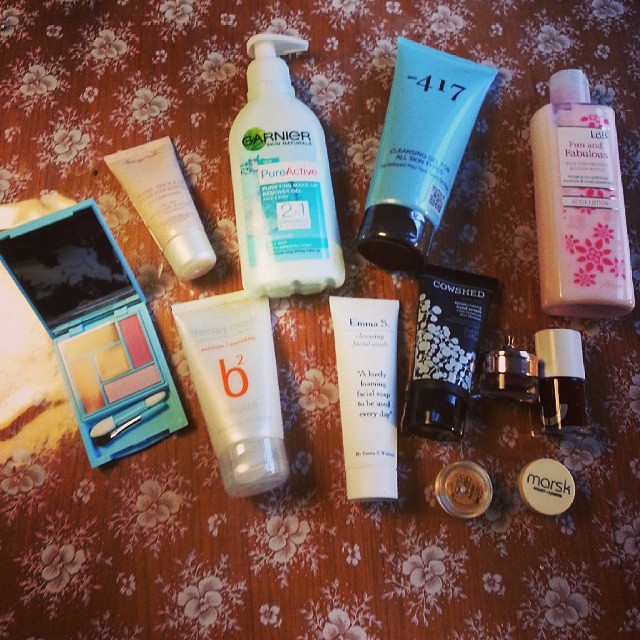The image showcases a collection of healthcare and beauty products neatly arranged on a surface that appears to be a reddish-brown floral-patterned blanket. The background features white flowers and leaf details, adding a touch of elegance to the display. The products are laid out from left to right, starting with a blue compact eyeshadow palette that includes two small applicator tools and a mirror. 

Next, there is a small bottle of hand lotion, followed by a slightly larger bottle of a similar product, presumably also a type of hand lotion. Among the array is a Garnier Pure Active product, likely related to hair care. Noteworthy is the 417 Cleansing Gel Foam, designed for all skin types, which is packaged in a blue container with a black twist-off lid. 

Additionally, the display includes a white squeeze tube labeled 'Emma S.', indicative of being a cream. A smaller black tube with the brand name 'Cow Shed' and a white design suggests a refined beauty product. Several tiny lip gloss containers are visible, alongside one that resembles a nail polish bottle. Rounding out the collection is a bottle of pink lotion adorned with floral designs and the word 'Fabulous,' hinting at a luxurious, fragrant hand or body lotion.